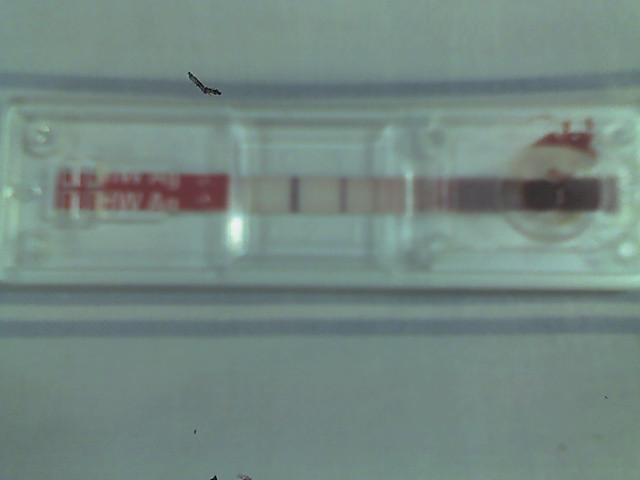A highly blurred photograph captures a scene with a gradient blue backdrop, transitioning from light blue at the top to a slightly darker blue in the middle. A black marking, reminiscent of a bird with outstretched wings, is positioned at the base of this darker blue section. Below this, a blurred white rectangle is visible, appearing to be a clear plastic tray divided into three segments. A horizontal band decorates the middle of the tray: the left segment showcases a white and red pattern, the center segment is white with two black lines, and the right segment displays a white and black design with a red and white circular motif. The overall background of the image is gray.